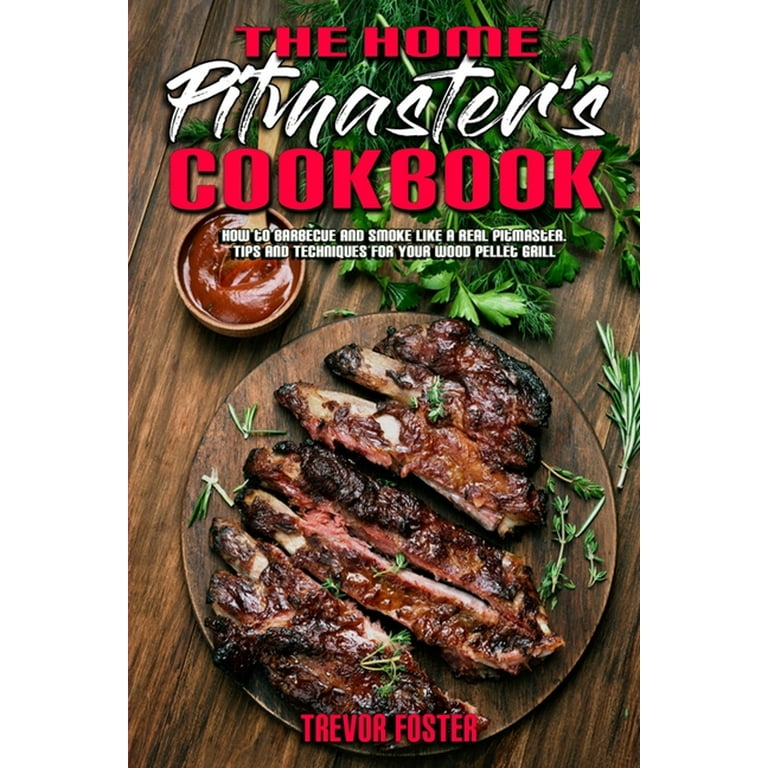The image is the cover of a book titled **"The Home Pitmasters Cookbook"**. The title is prominently displayed with **"The Home Cookbook"** in red text, and **"Pitmasters"** in a distinctive white and black script. Beneath the title, the subtitle **"How to Barbecue and Smoke Like a Real Pitmaster: Tips and Techniques for Your Wood Pellet Grill"** is clearly visible. At the bottom, the author's name, **Trevor Foster**, is printed in red. The cover features a tantalizing photograph of well-grilled ribs on a wooden plate, resting on a dark wood table. The ribs are garnished with rosemary sprigs and accompanied by a bowl of rich, amber-colored barbecue sauce with a wooden spoon. Additional garnishes, such as cilantro or coriander, are artfully scattered around the plate, enhancing the rustic presentation.